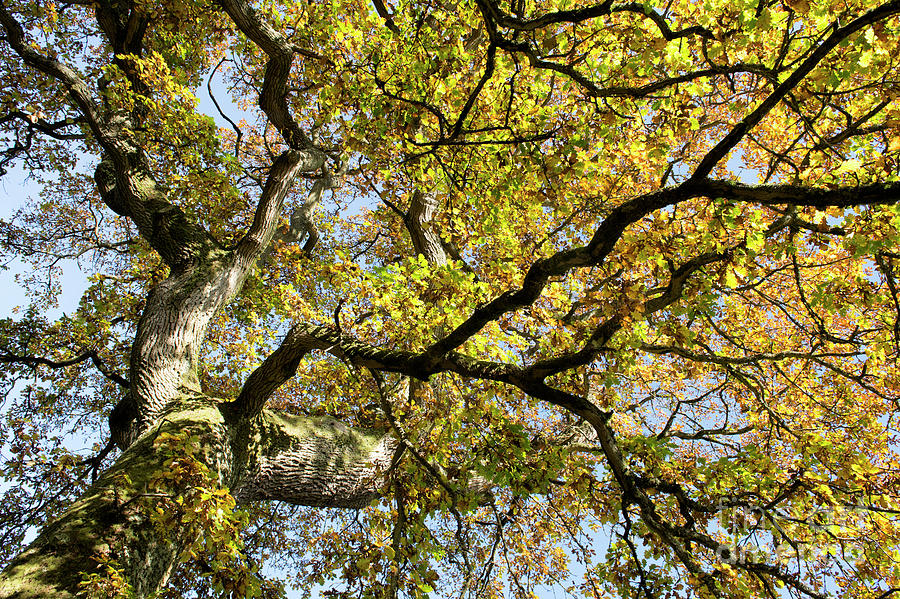This image depicts a towering, old oak tree, viewed from the base of its substantial trunk looking upward through its sprawling branches. The photo captures the visual impact of the tree's extensive canopy, which stretches across the entire frame, highlighted by the use of a wide-angle lens. The leaves on the branches showcase a vibrant array of fall colors, including lime green, yellow, orange, and brown, indicating the season is likely autumn. The lush green moss growing on the brown bark of the trunk adds a rich texture, adorned with some of the colorful leaves. Sunlight filters through the dense canopy, casting beautiful shadows and illuminating parts of the bark, which glows under the bright afternoon sun. The background reveals a clear, saturated blue sky, with no clouds visible, emphasizing the sunny day and enhancing the overall brilliance of the scene.